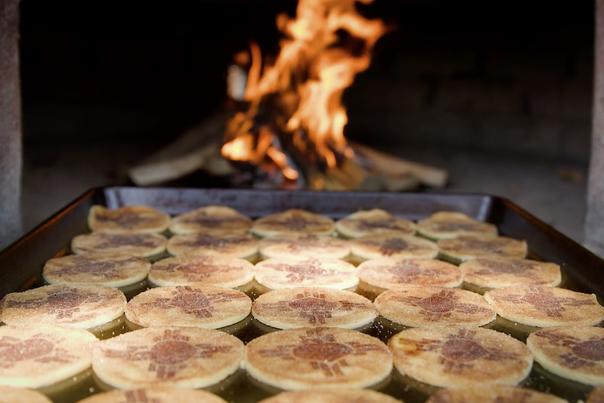The image depicts a rustic baking scene featuring a wooden log fire inside a brick oven. In the foreground, there is a metal baking sheet containing 30 round, flat items arranged in a precise 5 by 6 grid. Each item is light brown in color with symbols resembling a cross with a circle in the center, intricately patterned on the surface. The symbols appear to be red or brown in color, adding a decorative touch. The oven’s interior glows warmly from the fire, casting a cozy light on the baking sheet. The fire is fueled by wood, creating a traditional and inviting baking ambiance. The dark background contrasts with the bright flames and the neatly arranged baked goods, highlighting the artisanal and appetizing nature of the scene.